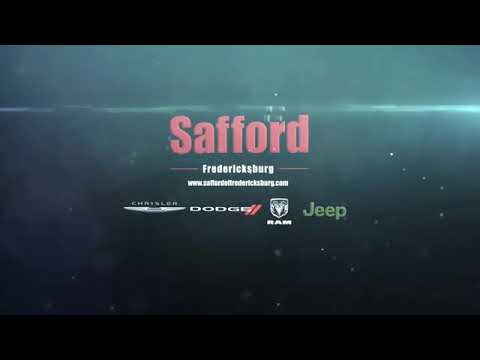The image appears to be an advertisement, possibly a screenshot, showcasing a dealership's promotional material with a dark, smoky blue background that evokes an underwater ambiance with small bubbles. Centered in the image in prominent, slightly faded red text is the word "Safford". Directly below, in smaller white text, is "Fredericksburg". Further down, there is a URL: "www.SaffordFredExpert.com", rendered in very small text. Following this are four automotive brand logos: Chrysler with its emblem, Dodge with distinctive red slashes over the "E", Ram with its iconic Ram's head symbol, and Jeep in dark green text. The advertisement is framed by black borders on the top and bottom, with a light streak cutting through horizontally, one-third from the top. Overall, this evokes the feel of an automotive dealership advertisement.